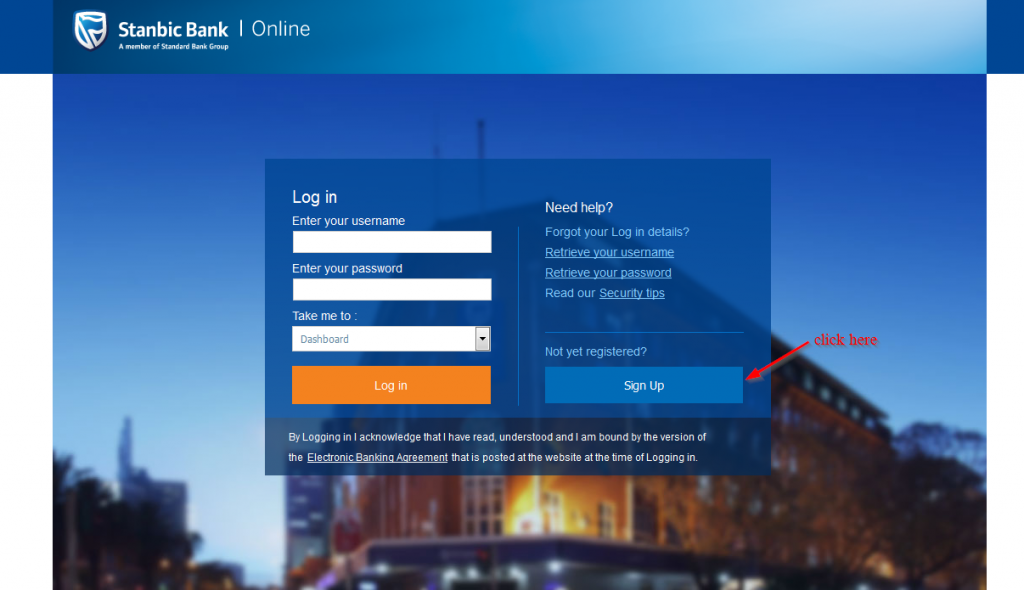The image depicts the initial login page of a website, predominantly colored in various shades of blue. The background features a scenic view of a building captured at sunset, with a few lights on inside while many remain off, adding a serene and slightly blurred effect to the backdrop. 

At the top of the page, a blue header showcases the logo of "Stan Bic Bank," a member of the Standard Bank Group, designed as a shield-emblem incorporating a flag, rendered in blue with a white outline. The text "Stan Bic Bank, a member of Standard Bank Group – Online" accompanies the logo.

Prominently featured in the center is a login box. Inside this box, instructions are provided to enter a username and password, with the option "Take me to" defaulting to the dashboard. Below these fields are two buttons: "Login" and another one labeled "Sign up," the latter marked with an arrow and red font that reads "Click here," guiding new users to register.

To the right of the login fields, within the same blue box, there's a series of help options in a neatly organized format. These include "Need help?", "Forgot your login details?", "Retrieve your username," "Retrieve your password," "Read our security tips," and "Not yet registered?"

At the bottom of the sign-in box, a disclaimer is present, stating, "By logging in I acknowledge that I have read, understood, and am bound by the version of the electronic banking agreement that is posted at the website at the time of logging in."

This detailed description encapsulates both the visual and textual elements of the login page, providing a comprehensive overview.